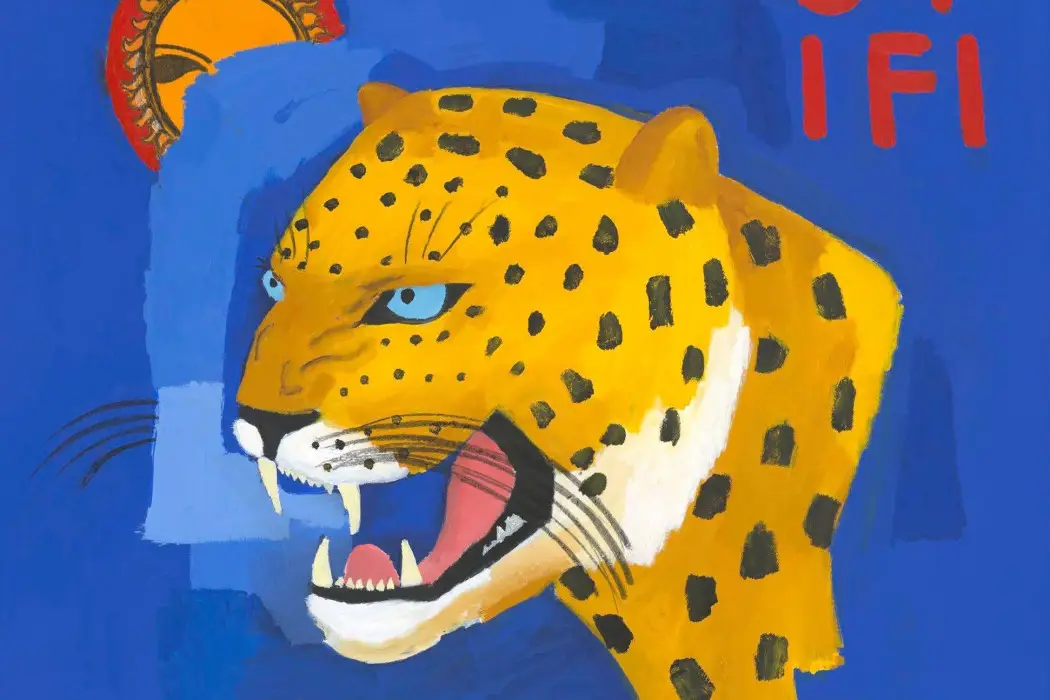This vibrant painting, possibly a watercolor, features the striking head and neck of an ornately detailed jaguar. The jaguar, an orangish-yellow with black spots, has white cheeks, a white underpart of its lip, and a white area beneath its nose. Set against a royal blue background, the jaguar's blue eyes and open mouth with a pink tongue and four prominent fangs—two on the top and two on the bottom—convey an intense, growling expression, further emphasized by its furrowed eyebrows. Long whiskers extend from the sides of its face. In the top left corner, partially obscured by a swatch of blue, is a stylized sun diagram with one visible black eye, encircled by a red halo. The top right corner prominently features the red lettering "IFI." The overall composition blends different shades of blue, adding depth and contrast to the jaguar and the surrounding elements.